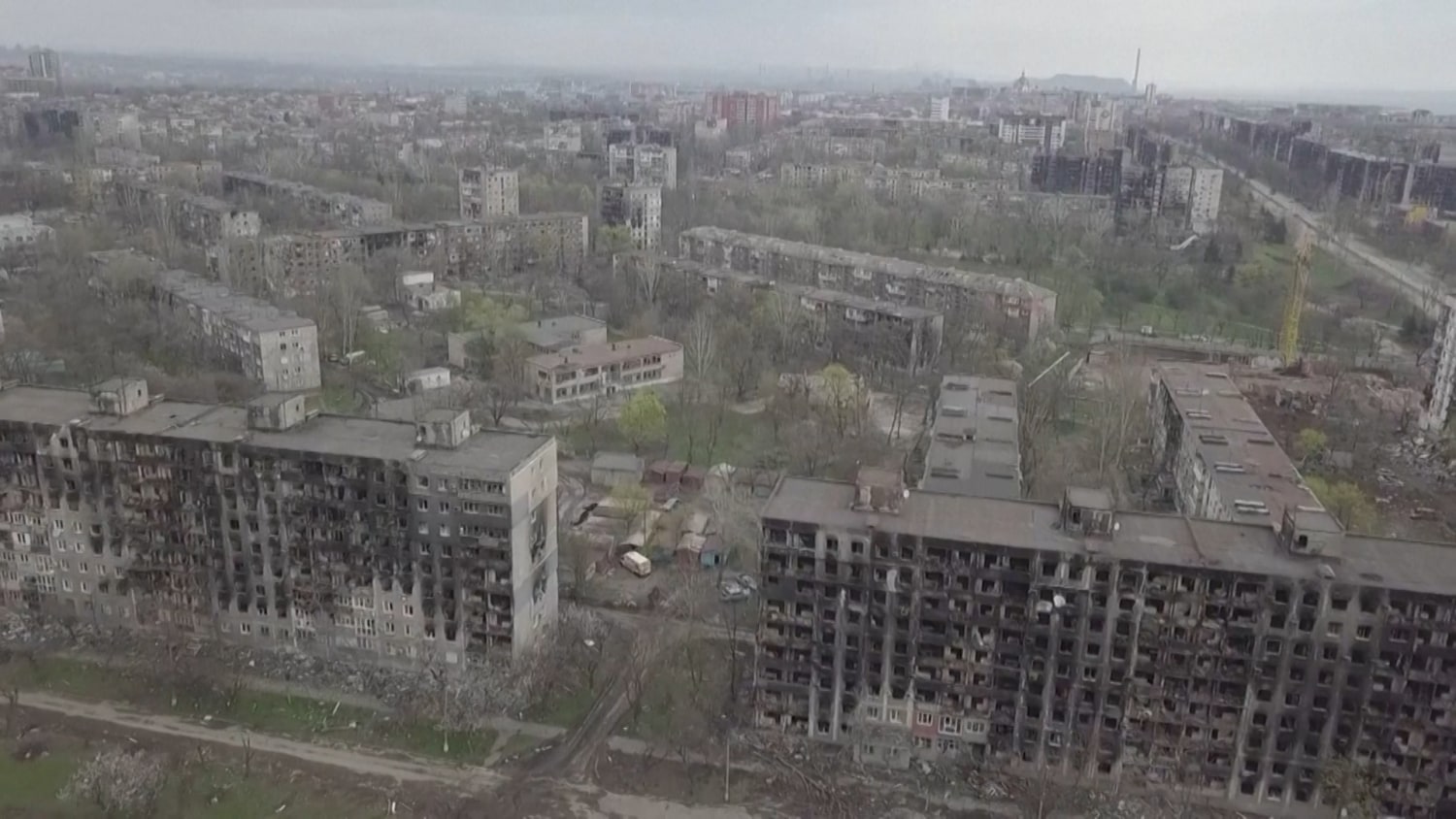An aerial photo, likely taken from a helicopter or drone, captures a city that appears to be in the aftermath of war, possibly in Chechnya. The image is of very low quality, with a gray, blurry sky dimly lighting the scene. The cityscape, dominated by concrete apartment buildings of varying heights, shows significant destruction. In the foreground, two large multi-story apartment buildings feature prominent black burn marks on the fronts and sides, with all windows blown out and debris scattered around. The remnants of a building that looks like it has been burned or bombed sit at the very front, with its facade collapsed, exposing the metal structure beneath. The background reveals a skyline with distant mountains, interspersed with patches of tree growth and bushes. A bridge is faintly visible in the right-hand corner, further adding to the sense of a devastated urban area.